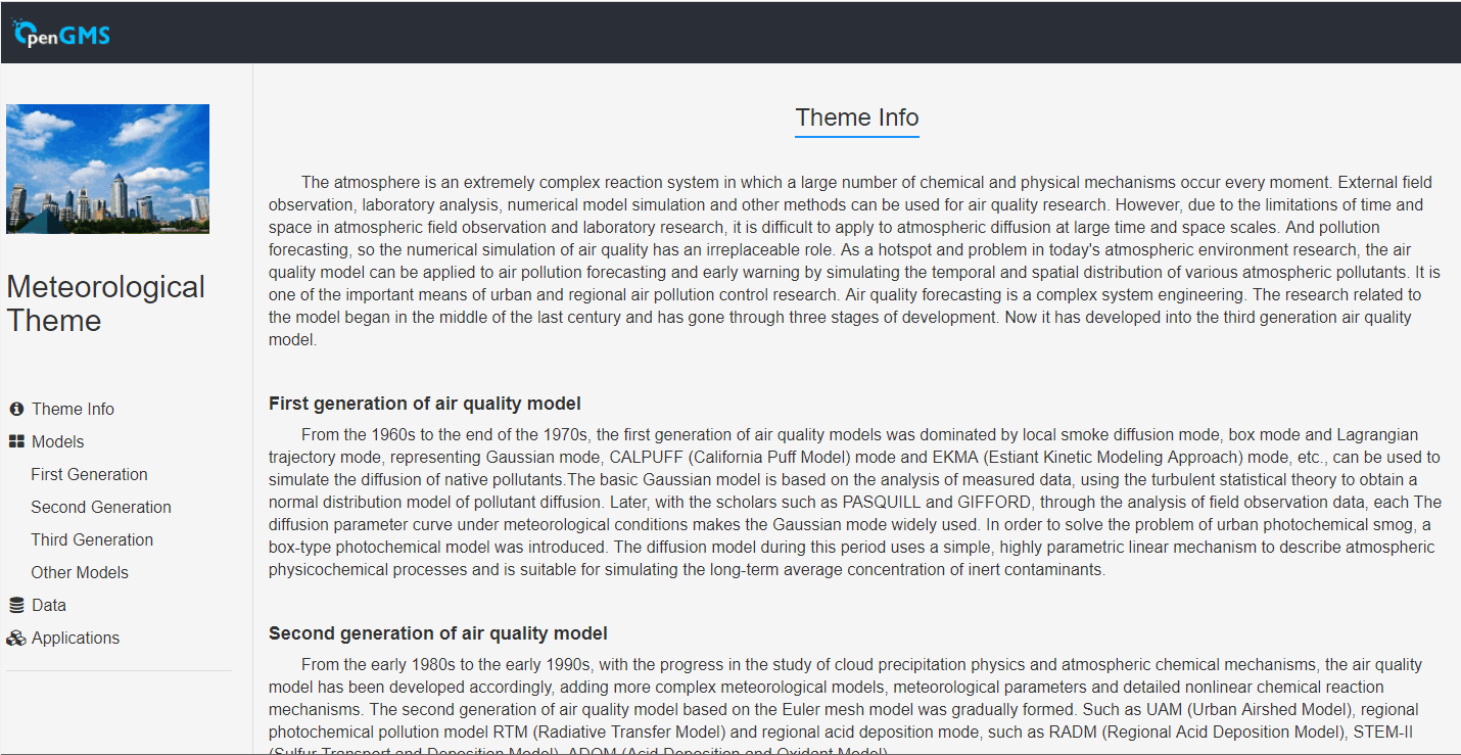A screenshot of a website named OpenCMS is displayed on the desktop. The website details various themes, with a focus on musical and meteorological themes. The specific theme highlighted in this screenshot is the "Meteorological Theme." This theme is designed for use with a green screen effect, allowing users to create the illusion of standing in front of a city skyline with clouds and a clear sky passing by.

The page provides comprehensive information about this theme, including descriptions of first, second, and third-generation models. It explains how each generation can be utilized to enhance the visual effect of a clear day in the city. Additionally, the page covers background information on relevant air quality models, specifically mentioning a model referred to as "cow puff."

Overall, the OpenCMS website serves as a resource for users looking to incorporate various themes into their presentations, particularly those related to weather and background effects. The detailed descriptions and guidelines provided help users make informed choices about which themes to use for their specific needs.